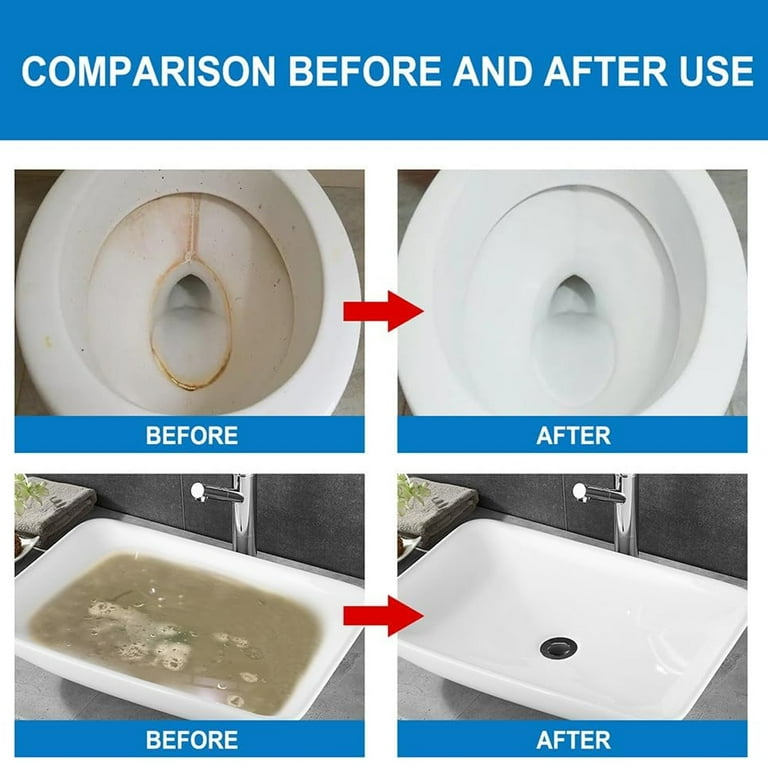This advertisement for a powerful cleaning formula showcases its impressive effectiveness on ceramic surfaces. At the top, a light blue banner with white lettering reads "Comparison: Before and After Use." Below it, a set of four images detail the transformation. On the top left, a toilet bowl exhibits a dirty, brown ring of filth surrounding its center. Below this, a blue banner with white lettering reads "Before." A red arrow points to the top right image, where the toilet bowl gleams spotlessly clean. The "After" label is also displayed in a blue banner with white lettering. 

The bottom set of images follows a similar layout. On the left, a white sink is filled with murky, gray, and black water, against a backdrop of a gray wall and a silver faucet, with a brown towel in the upper left corner. The "Before" label is seen again in a blue banner with white lettering. A red arrow leads to the right, showing the same sink now pristine, with clear visibility of the black drain and free from any dirty water. This "After" image also features a blue banner with white lettering.